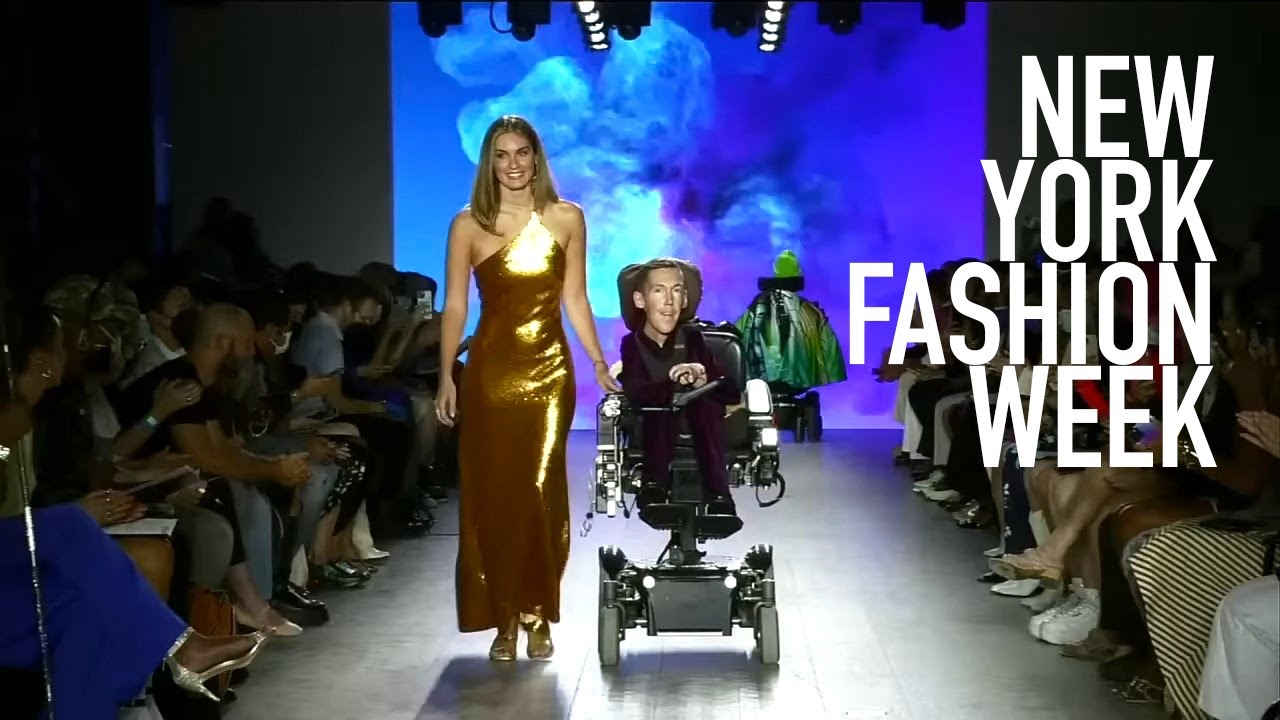Captured during New York Fashion Week, this image showcases a runway scene in vibrant hues of gray, blue, light blue, and purple, with a swirling pattern adorning the background. An audience frames the space on either side. The focal point is a diverse pair of models: a stereotypical blonde-haired model in a shimmering gold dress that elegantly drapes to her feet, baring one shoulder with its asymmetrical one-strap design, strides confidently down the runway. Beside her, a well-known TikTok or YouTube personality, a physically disabled man, navigates in a sophisticated, custom-designed motorized wheelchair, reminiscent of those used by Stephen Hawking due to his severe scoliosis or degenerative illness. He is dressed in a deep burgundy dress shirt and slacks, accented by a black vest. In the backdrop, another model, also using a motorized wheelchair, exits the stage. The entire setup is framed by text in white sans serif font stating "New York Fashion Week" on the right-hand side. A mysterious green object with a covering and a green ball adds an additional note of intrigue behind the models.